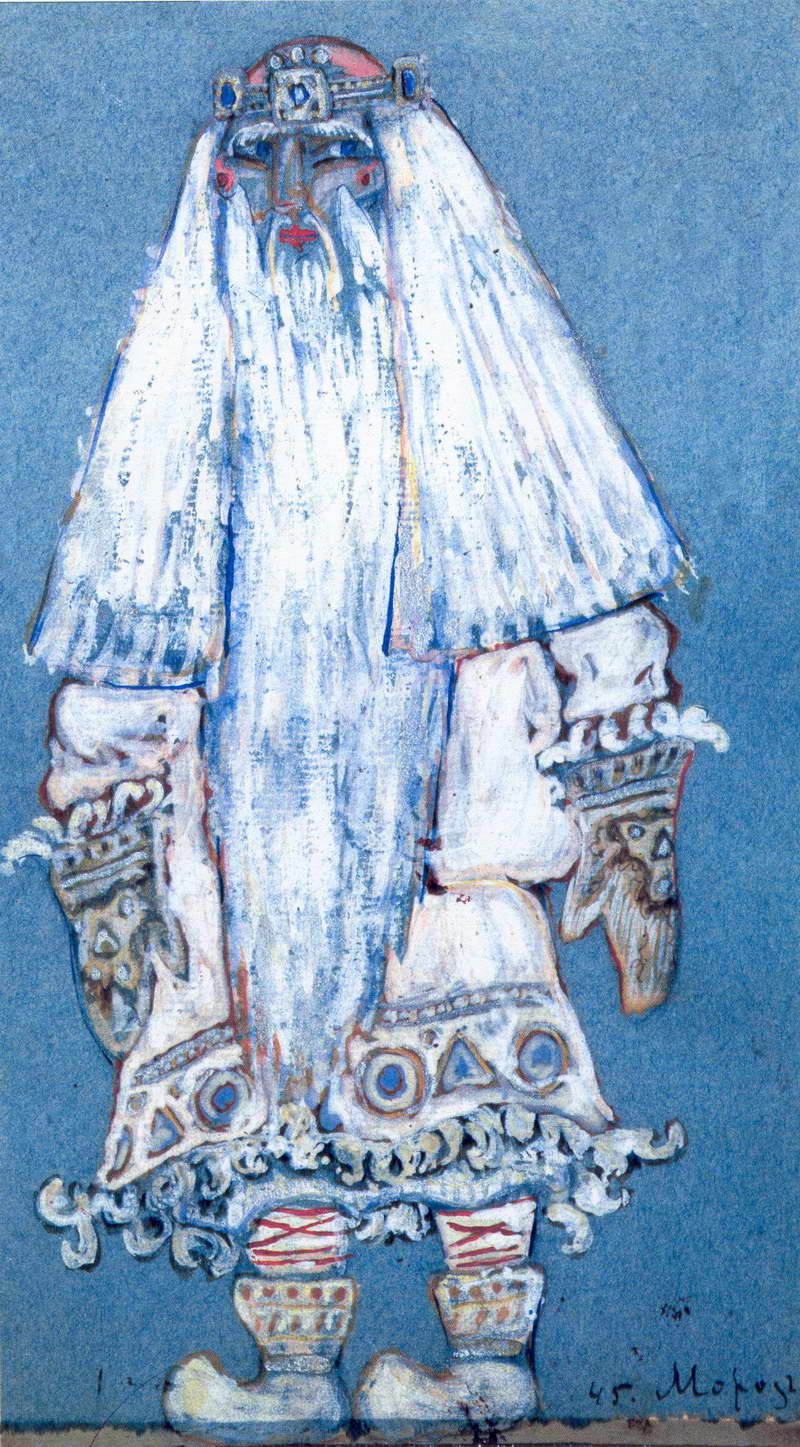This painting depicts an ancient figure, possibly a Mongolian warrior or king, set against a striking blue background. The central character is richly adorned in a predominantly white ceremonial robe that features intricate designs. Prominent blue and white hues define the overall color scheme. The man, who exudes an air of contemplation, is distinguished by his exceedingly long white and blue beard that extends past his knees, and his equally long hair that cascades past his shoulders. Atop his head rests a crown adorned with blue jewels and a red top, contributing to his regal appearance.

His face is partially masked with red and gray, accentuated by red dots on his cheeks and red lips, with visible details of his nose and lips suggesting a deeply thoughtful demeanor. His hands are encased in ornate gloves with elaborate designs, while his socks, decorated in blue and red patterns, peek out from under the robe. Footwear resembling traditional Mongolian boots, crafted from a mix of cloth and leather with upturned tips, completes his attire. The painting is signed by the artist in the lower right-hand corner, with the signature starting with "M-O-H-E-Y" and the number "45" displayed prominently.